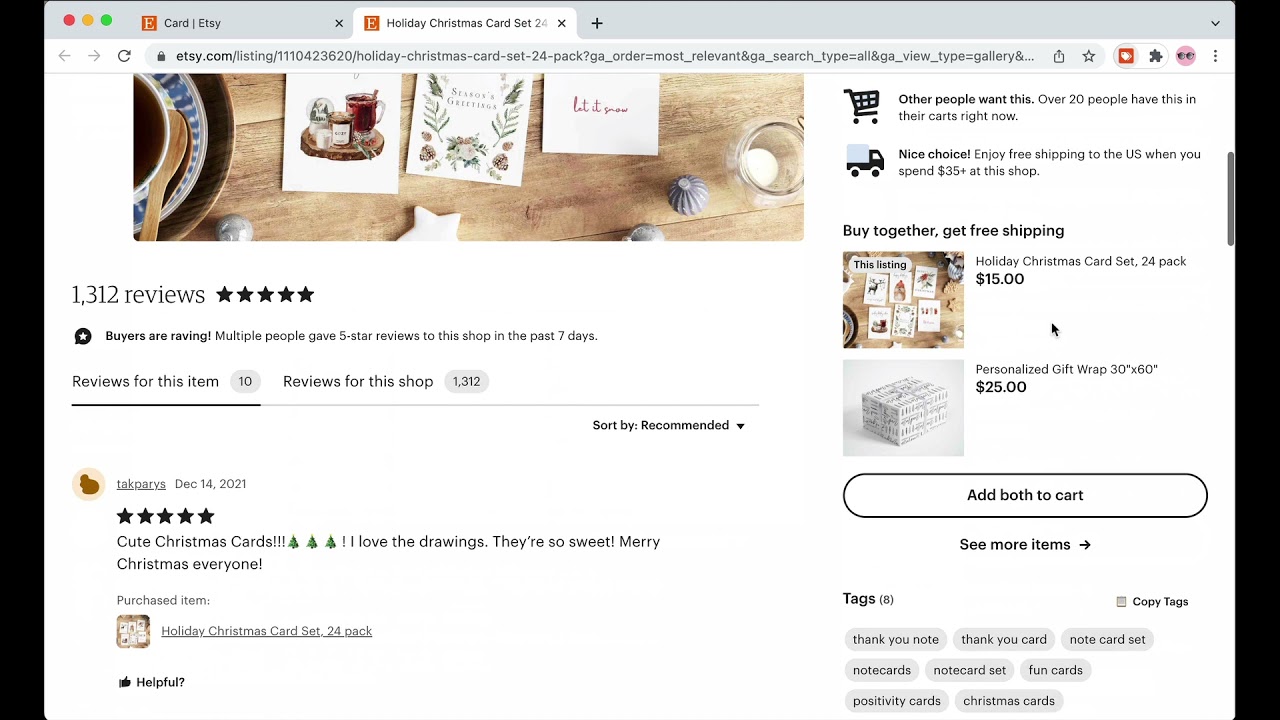This screenshot captures a detailed view of a results page on the Etsy website. In the top left-hand corner, the Etsy logo and name are prominently displayed, along with a search box at the top of the page containing the query "holiday Christmas card set 24." The results for this search are now being displayed on the site.

At the top of the page is an aesthetically staged photograph showcasing a set of Christmas cards arranged on a rustic wooden table. The scene is adorned with small, glowing candles and a cozy coffee cup, adding to the festive ambiance.

Beneath the photograph, a series of reviews highlight the popularity of these cards, which have an impressive five-star rating. One written review is particularly enthusiastic, praising the cards' delightful illustrations and extending warm holiday wishes: "Love the cards, love the drawings, they're so sweet, Merry Christmas everyone."

On the right-hand side of the page, several functional elements and additional features are visible. There's a shopping cart icon and information about potential free shipping offers for bulk orders. Additionally, there are suggestions for personalized gift wrap that complements the Christmas cards, enhancing the overall shopping experience.